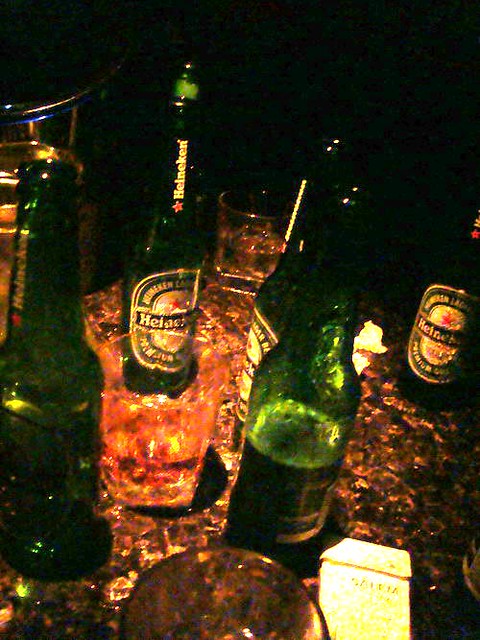This image captures a dimly-lit bar scene, focusing on a medium to dark brown table covered with an assortment of drinks and items. Central to the scene are five green Heineken beer bottles with visible logos, some partially drunk. Alongside the beer bottles are three shorter whiskey glasses filled with various amounts of liquid, one containing a white straw. In the top left corner sits a silver ice bucket with a thin handle. The tabletop also holds a pack of cigarettes with unreadable text, possibly due to the poor lighting. There's also some indistinct paper or trash scattered across the surface, adding to the casual and cluttered ambiance. The background remains obscured, suggesting the photo was taken at night with inadequate lighting.